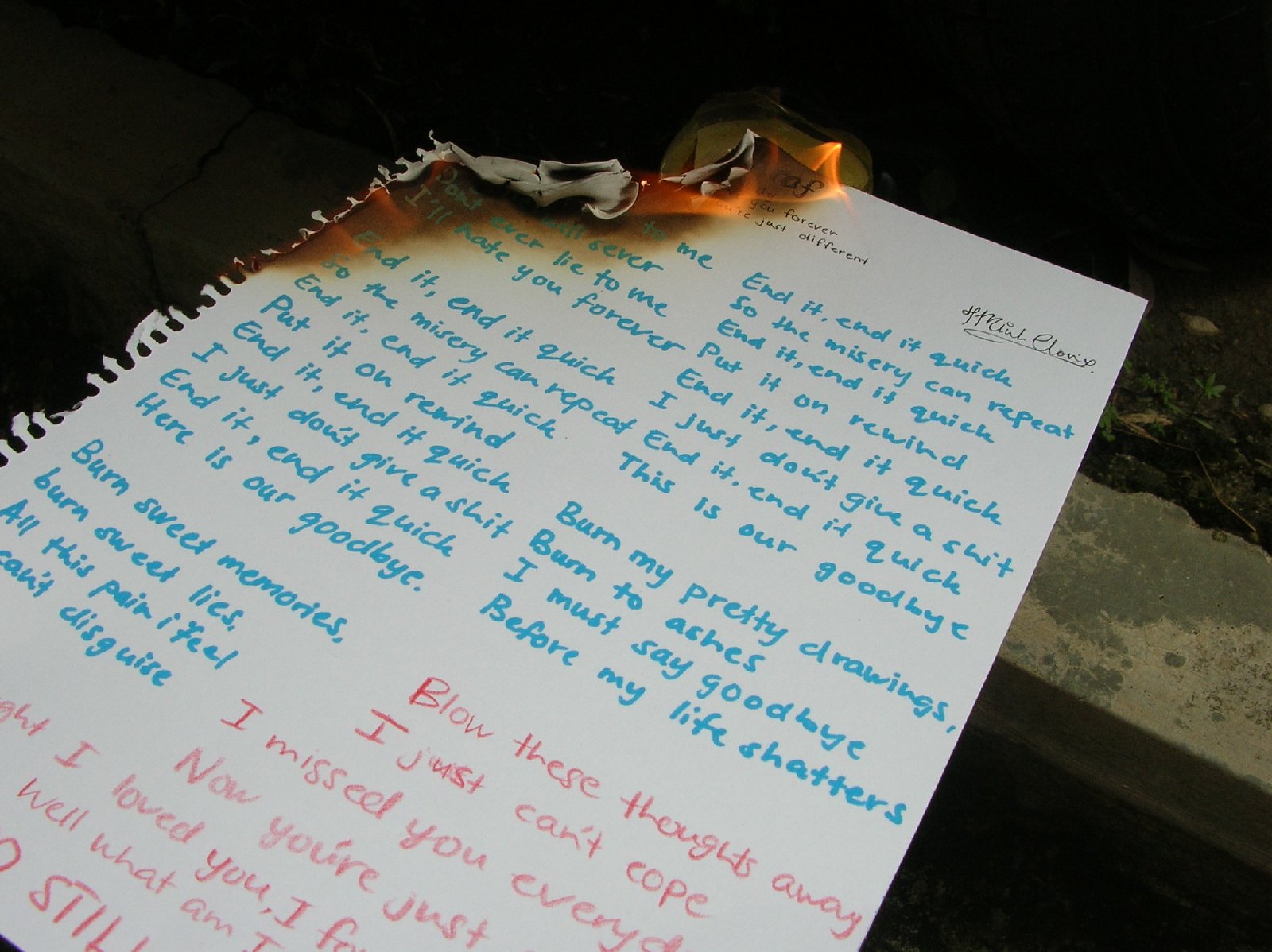The image displays a piece of notebook paper, slightly charred and curling from orange flames consuming the top left corner. The paper features an extensive handwritten poem predominantly in blue ink, with particular emphasis on recurring, anguished phrases such as "end it, end it quick," "put it on, rewind," and "I just don't give a shit." Lines like "never lie to me, hate you forever," and "burn sweet memories, burn sweet lies," convey pain and betrayal, mingling with verses about finality and loss. At the top right, a small, cursive black ink signature, difficult to decipher, is visible. Across the bottom right, interspersed red text, akin to crayon, disrupts the blue text's rhythm with sentiments like "blow these thoughts away" and "I miss you every day, now you're just...," before the image cuts off. The photograph, taken in a dimly lit outdoor setting near a concrete garden barrier, captures the intense emotional turmoil reflected in the burning, poetic words.